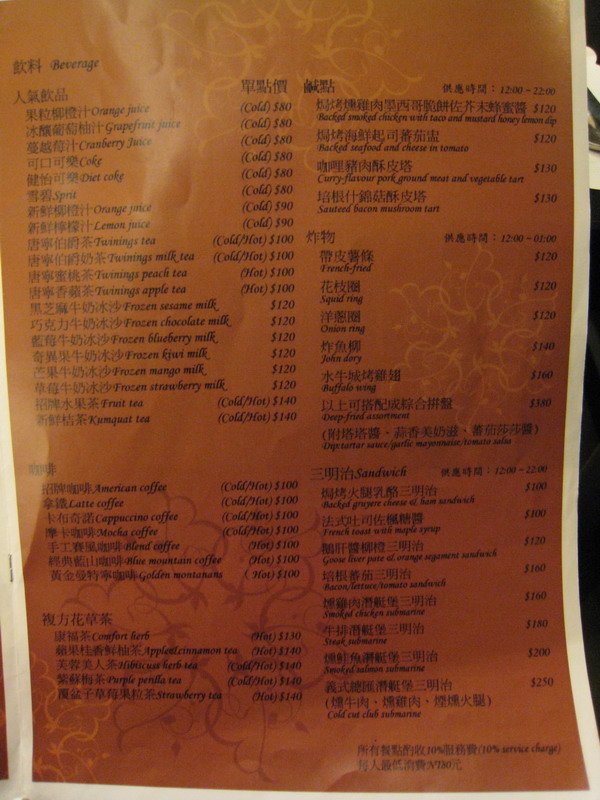Here we have an intricately designed menu printed on brown paper with white edges. The text is primarily in Chinese, featuring black ink for clarity. At the top, the heading "Beverage" is written in English. The menu includes a variety of drinks such as orange juice, grapefruit juice, cranberry juice, Coke, Diet Coke, lemon juice, and several types of teas, including a specific offering labeled as "Tammings Milk Tea." Additionally, it lists coffee options like latte and a special "comfort blend." 

The menu is adorned with subtle artistic touches; delicate drawings in a light brown hue are visible in the background. At the top, these illustrations resemble miniature people, adding a whimsical touch. Towards the bottom, there are faint outlines of various characters, which look like small balloons floating in the air, contributing to the overall charm and aesthetic appeal of the menu. Large prices for the items can be seen, ensuring easy readability for customers.